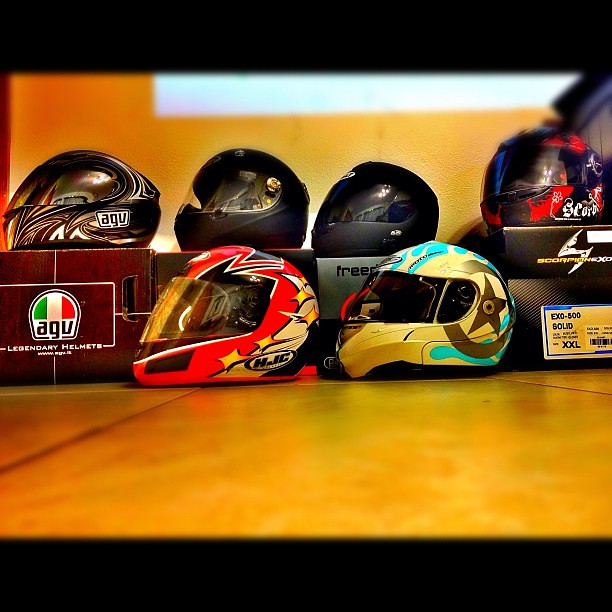This photograph captures six intricately designed helmets, meticulously arranged in a store display case that is illuminated to give a golden hue, though the case itself might be white. The display is set against an orangish-brown wooden floor and matching wall background.

On the top row, from left to right, the first helmet is metallic with a swirl of red, white, and black, marked with the letters "A-G-U." Next to it, centered, are two black helmets: one accented with gold tracing and the other with blue detailing. The helmet on the far right of the top row is an eye-catching multicolored piece, predominantly black with red and blue designs.

The bottom row features two helmets directly on the store shelf. The one on the left is mostly red, adorned with blue and gold accents, and possibly labeled "H-I-C." Finally, the helmet on the right is striking with its blue and gold design, featuring a prominent gold star encased in a circle on the side.

Each helmet has a protective glass or plastic covering over its face area, adding to the pristine display of these vibrant and detailed items.